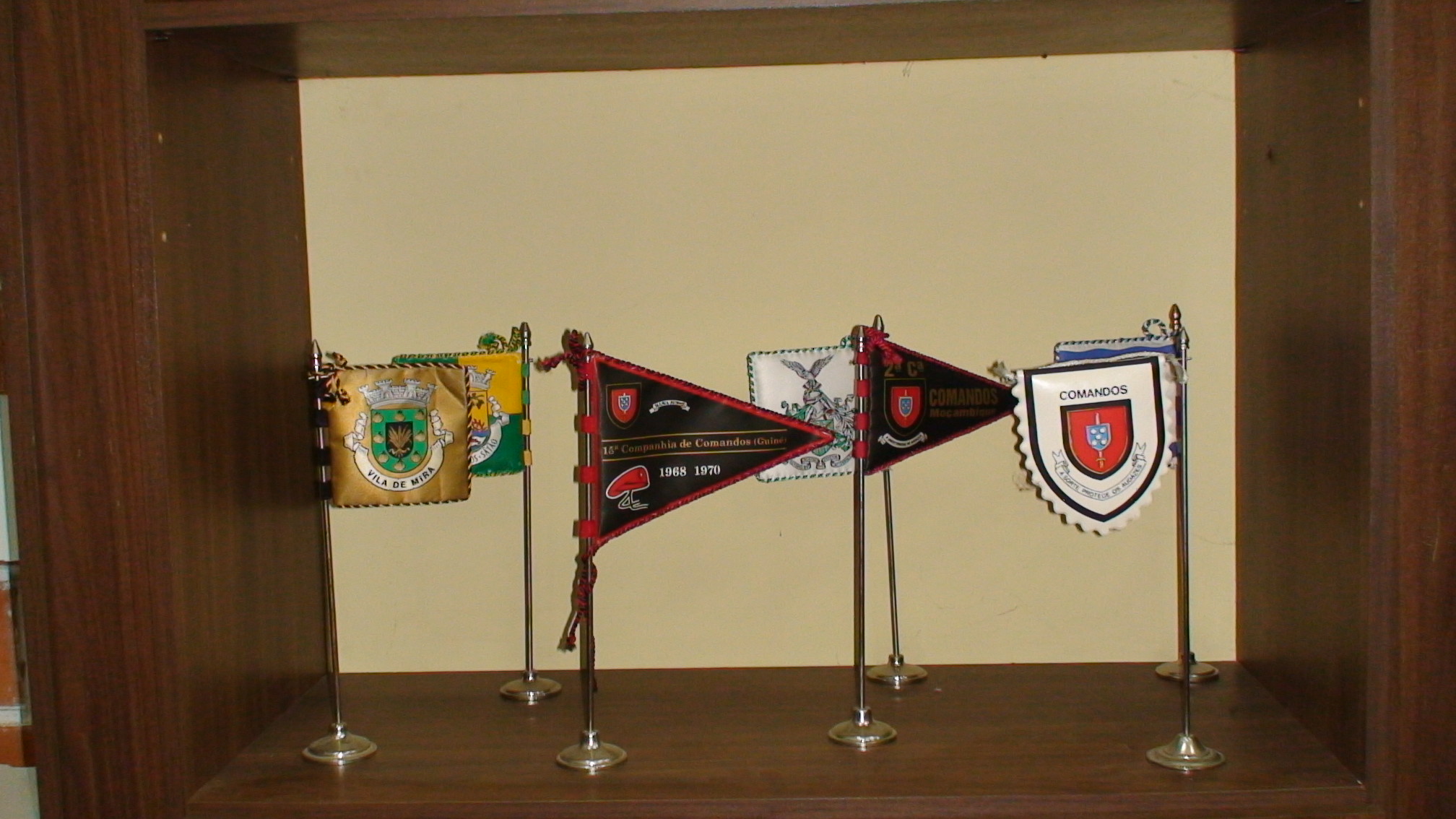In this detailed photograph, a wooden cabinet against a white or tan wall showcases seven different flags, each mounted on silvery metal poles with circular bases. The flags vary in shape, size, and design, representing different organizations or businesses. Starting from the left, the first flag is rectangular with a gold background and reads "Villa de Mira." Adjacent to it is a partially visible green and gold checkered flag. The third flag, a triangular one, marks the years "1968-1970", while the fourth flag features a white background possibly depicting an eagle. To its right, another triangular flag displays the word "Commandos." The next flag has a white background with a red shield, also inscribed with "Commandos" at the top. The final flag is mostly concealed, showing hints of white and blue. These diverse flags, captured against the backdrop of the wooden cabinet with a paneled wall, create a vibrant and organized display.